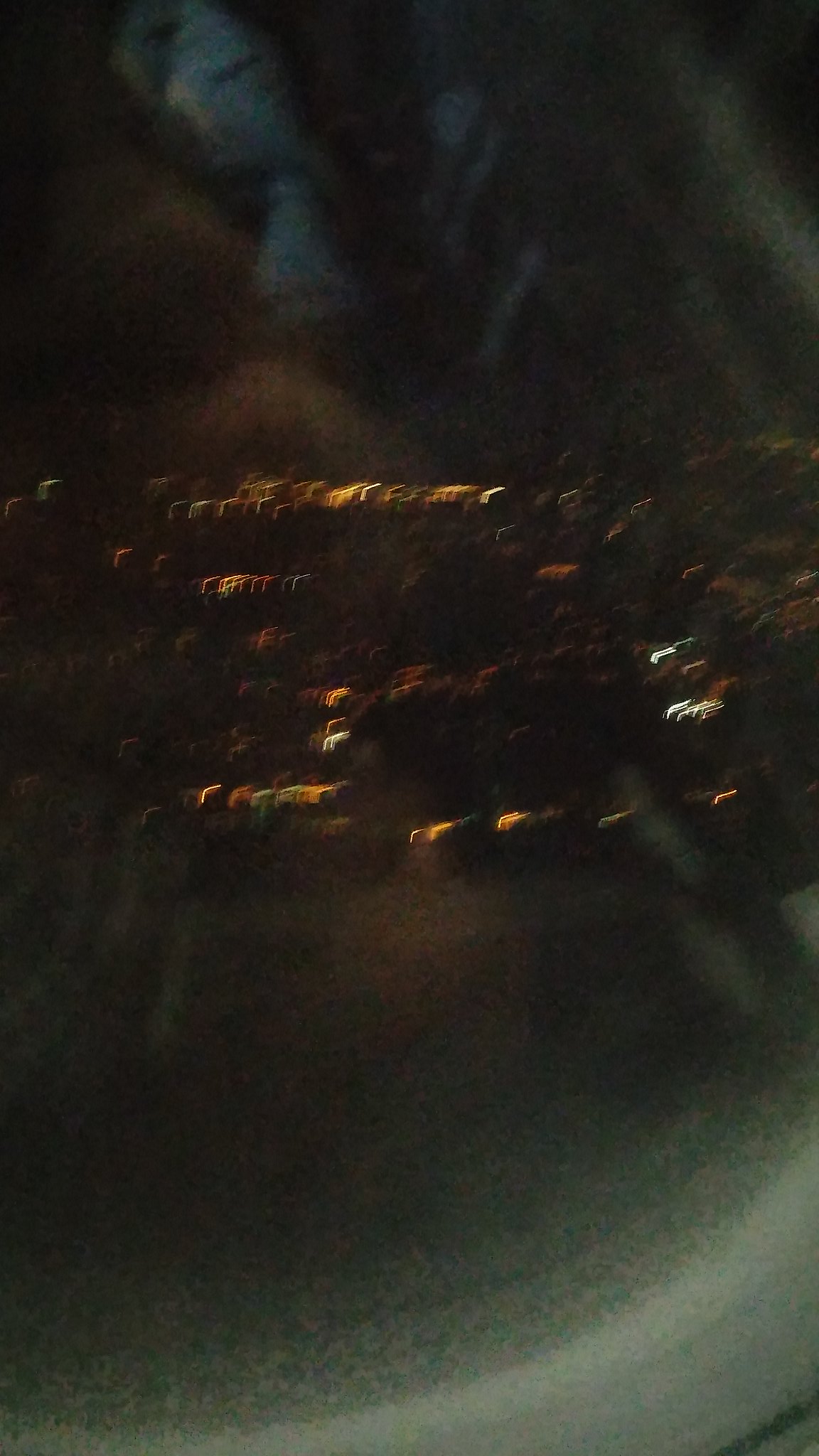This nighttime photograph, shrouded in blurriness and taken from what appears to be the window of a plane or helicopter, captures a cityscape bathed in various hues of lights. The scene features a collection of buildings and houses stacked closely together, emitting warm yellow and orange glows with occasional reds and greens. These light blobs, although indistinct, align in rows suggestive of a residential area. The window's edge, curving slightly upward to the right, along with the bottom third's gray and white borders, frame the image. Subtle reflections of the photographer, perhaps just peach splotches indicating hands or a portion of their face, further obscure the view. The image hints at trees and an expanse of grass bordering a possible road in the gray-blue segment at the bottom. Despite the movement and the window's reflection complicating the clarity, the overall impression evokes a bustling town lit up against the night sky.